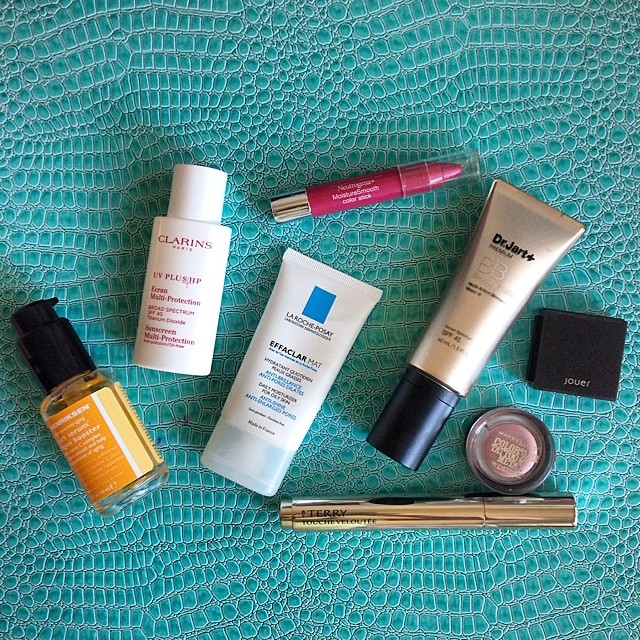A stunning flatlay of various makeup and beauty products is arranged on an eye-catching teal background that mimics the texture and appearance of alligator skin, with small, detailed scales. At the top center, a pink Neutrogena MoistureSmooth Color Stick with a silver end and clear cap stands out. To the right, a gold tube of Dr. Jart+ SPF 45 cream is capped in black. Nearby, a sleek black box with "JOUER" elegantly inscribed on it catches the eye. A circular clear container houses a vibrant purple powder, marked "Maybelline Color Tattoo Metal." Adding to the variety, a gold, mascara-shaped container branded "TERRY" lies nearby. On the left side, a clear bottle with a black pump features an orange label bearing the name "Henriksen." Below, a white bottle with a matching cap and label printed in red text reads "Clarins Paris UV Plus Broad Spectrum SPF 40 Sunscreen Multi-Protection." Finally, at the center, a white tube with a clear cap labeled "La Roche-Posay Effaclar Mat Hydratant" promises anti-shine and anti-balance benefits.